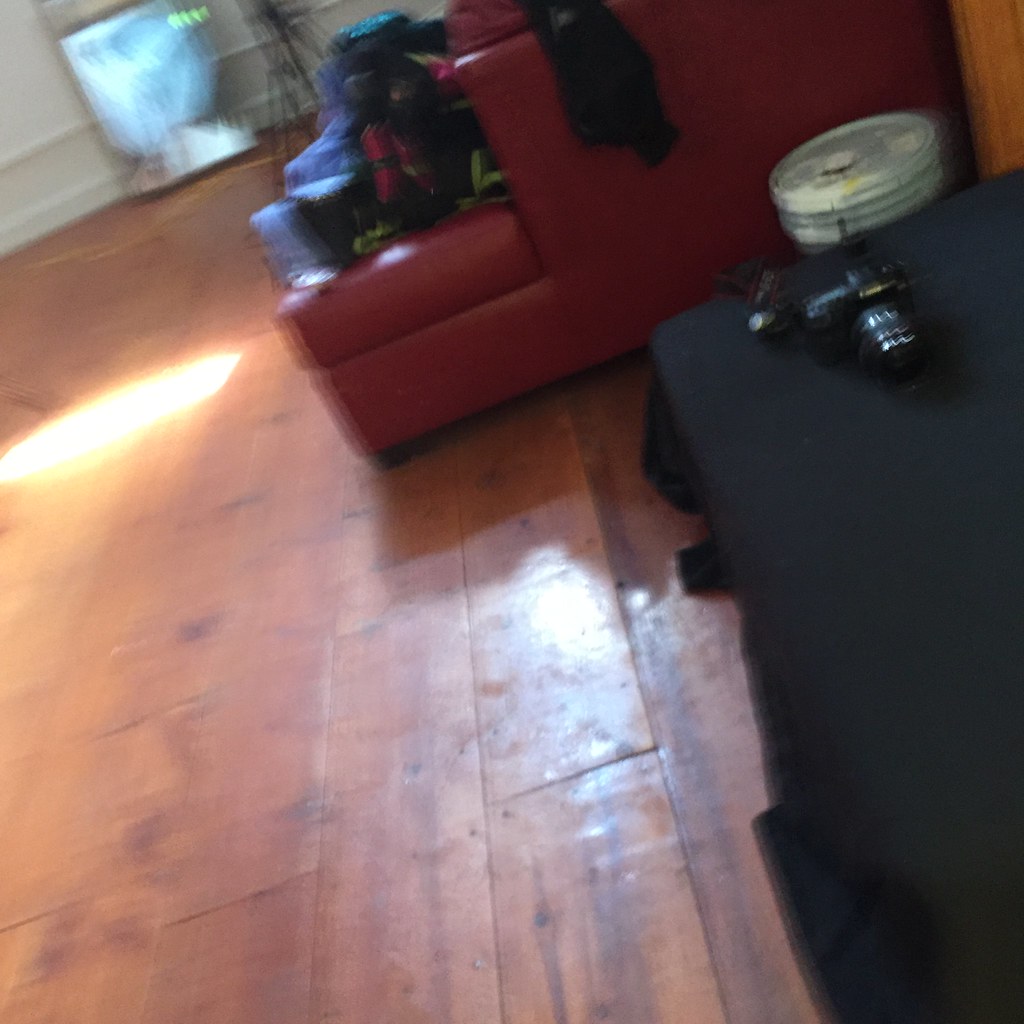This indoor photograph taken from a slightly elevated angle and tilted slightly to the right, showcases a detailed scene of a living room area. Dominating the foreground is a light-colored, large planked hardwood floor, with a distinct circle of sunlight illuminating the middle left side. To the right, a small table is covered with a black sheet, atop which rests a Canon camera at the end. Behind this table is a large gray plastic bucket, resembling a paint bucket. Directly behind the bucket is a red leather couch, noticeably draped with clothes and a shirt hanging over its arm.

To the upper left, a silvery object, possibly a bin, is visible with sunlight reflecting off the floor. In the far background against a white wall, several tripods and a light fixture are set up, adding a hint of a professional setting. A noticeable feature in the backdrop includes a white box with a blue light shining brightly from within it. The overall composition captures a mix of household and potential studio equipment, blending casual living space with technical elements.